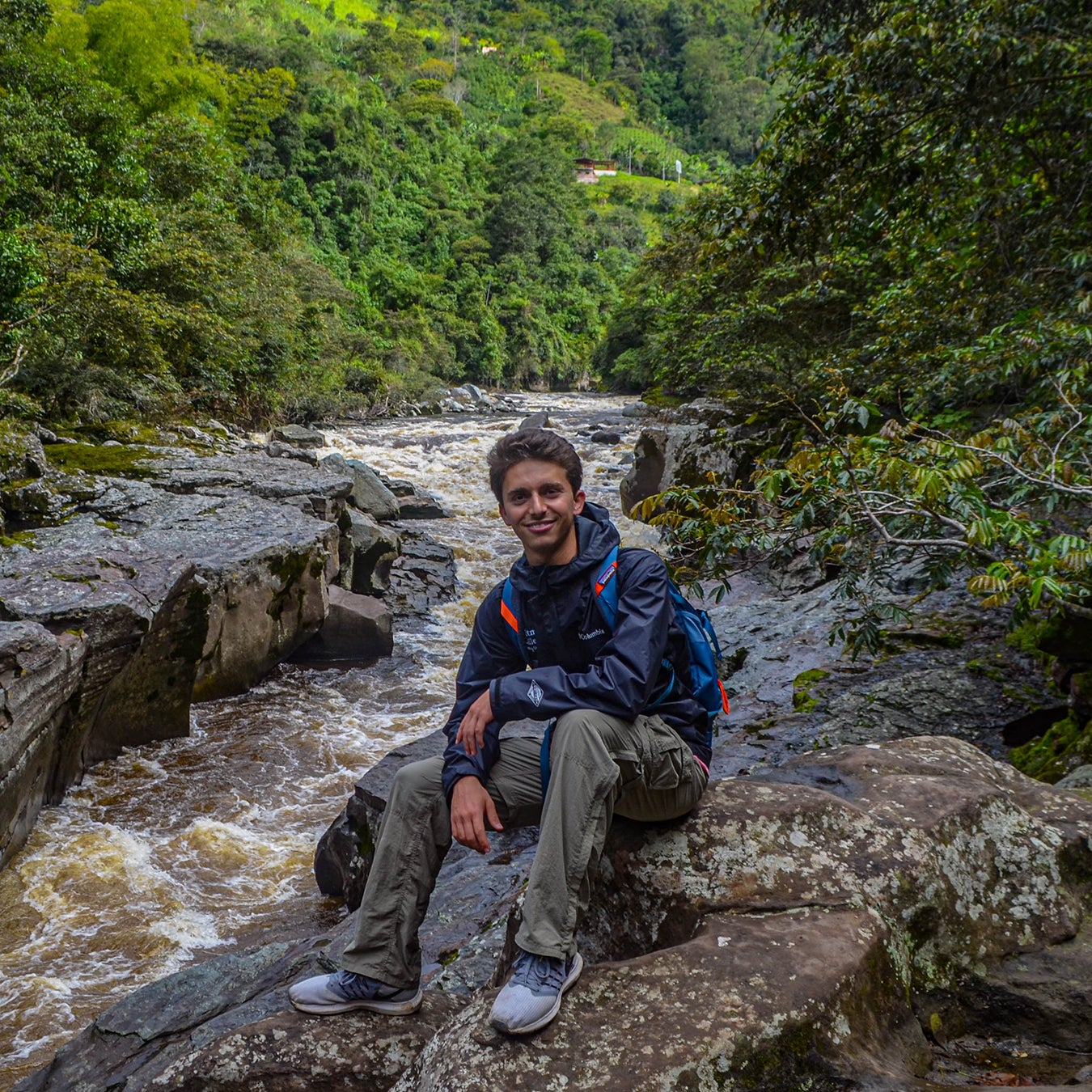The photograph captures a young man, likely in his late teens or early 20s, sitting on a dark gray, almost black rock formation covered with brown moss and lichen. He is smiling warmly at the camera, showcasing his short brown hair with a slight curl. Dressed for a hike, he's wearing a navy blue windbreaker or waterproof jacket with a hood, grayish cargo pants, and blue hiking trainers with pale gray and blue accents. A bright blue and neon orange backpack rests against his back, adding a pop of color to his outdoor gear.

Behind him, a fast-flowing, dirty brown river with whitewater rapids cuts through the rugged landscape. Rocks jut out on either side of the river, which gushes vigorously around the formation he is perched on. The scene is enveloped by a lush forest with various types of trees in multiple shades of green. In the far background, almost obscured by the dense foliage, there appear to be some small buildings or houses, hinting at a remote hiking trail.

The overall atmosphere of the photograph is one of serene beauty and rugged natural charm, capturing the essence of a wilderness adventure in a mountainous area.